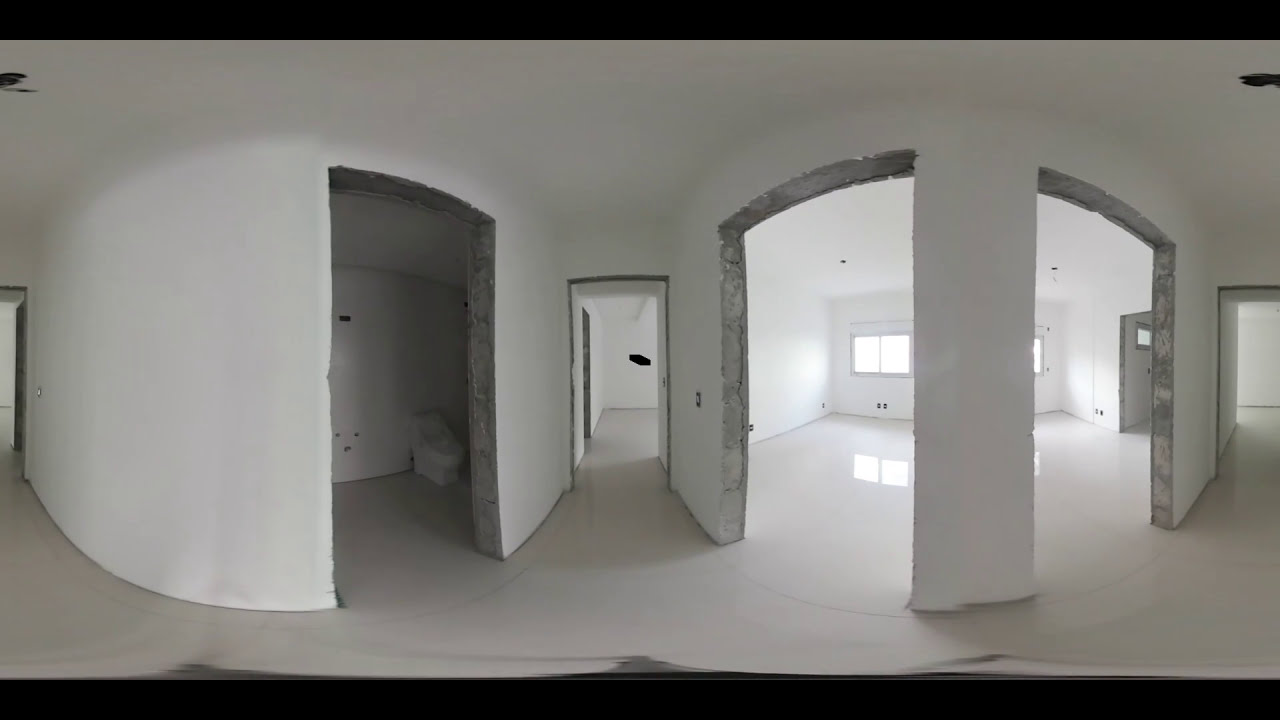This panoramic, 360-degree image showcases an interior space of an unfinished house, predominantly painted in white. The room appears jagged and rough, with exposed wall material and absent door frames, suggesting ongoing renovations. At the center of the image, a doorway leads into what appears to be a bedroom. To the left, a rough doorway opens to a bathroom that lacks lighting but houses a visible white toilet. The walls and ceilings curve, creating a bubble-like effect common to fisheye lenses. Moving right, there are two additional doorways, potentially leading to the same or different rooms, accompanied by a reflective, shiny floor that suggests tile material. Further right, an arched opening reveals a large, bright room illuminated by sunlight streaming through its windows. Additionally, a hallway extends to the right, contributing to the expansive and interconnected feeling of the unfinished living space.